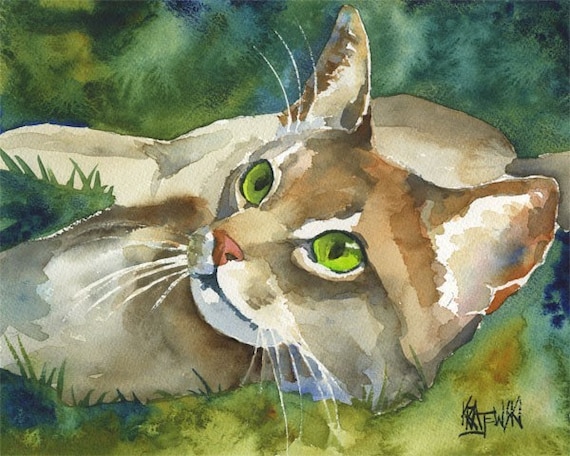This photograph captures a stunning watercolor painting of a cat in a relaxed pose. The cat lies on its side with its legs splayed out, head lifted slightly, and its gaze directed upward, seemingly entranced by an unseen object, perhaps a tree. The background is an abstract blend of greens and yellow greens, skillfully created by the artist through fluid, bleeding brushstrokes. The feline itself is rendered in various shades of tan, adding depth and texture to its fur, while its bright, glowing green eyes stand out vividly, drawing the viewer's attention. The contrast between the cat's detailed depiction and the abstract, verdant background creates a captivating and harmonious composition.